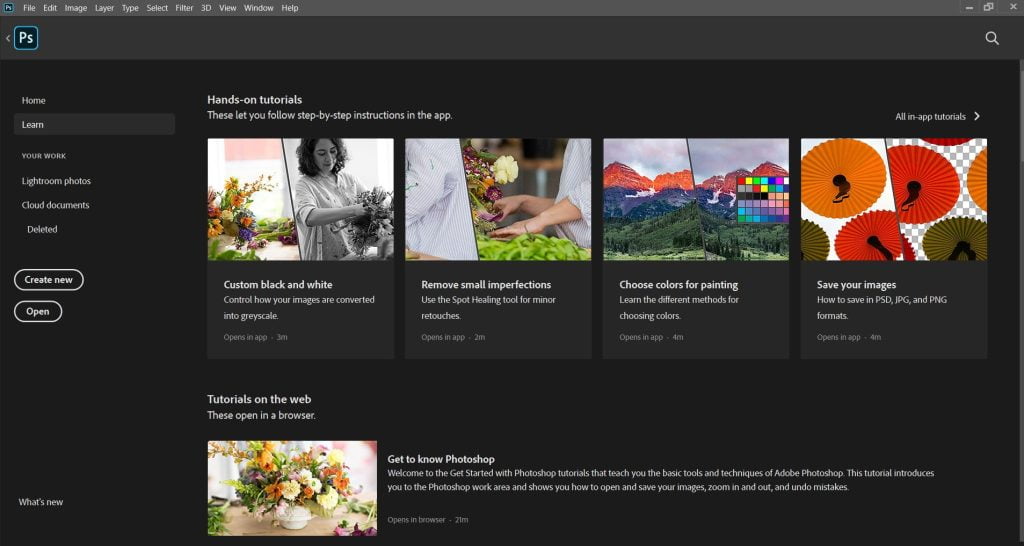A screenshot captured from within Adobe Photoshop, showcasing the interface in a horizontal rectangular frame with a black background. In the top left corner, the iconic gray-outlined PS logo in black signifies the presence of Photoshop. The top gray bar displays the menu options: File, Edit, Image, Layer, Type, Select, Filter, View, Window, and Help. 

On the left-hand side, the options are listed in white text against a black background: Home, Learn, Your Work, Lightroom Photos, Cloud Documents, and Deleted. Below these options are two oval buttons, the first one larger and labeled "Create New," and the second smaller one labeled "Open."

The right side of the screen features a row of tutorial images under the heading "Hands-On Tutorials." These include:
1. "Custom Black and White" with a relevant image,
2. "Remove Small Imperfections" with an appropriate example,
3. "Choose Colors for Painting" with a demonstrative image,
4. "Save Your Images" with a corresponding illustration.

Additionally, there are image tutorials accessible on the web, indicated by a picture of a white vase filled with a lush, colorful bouquet of flowers. To the right of this image, under the title "Get to Know Photoshop," there is a paragraph providing more detailed information about Photoshop's capabilities.